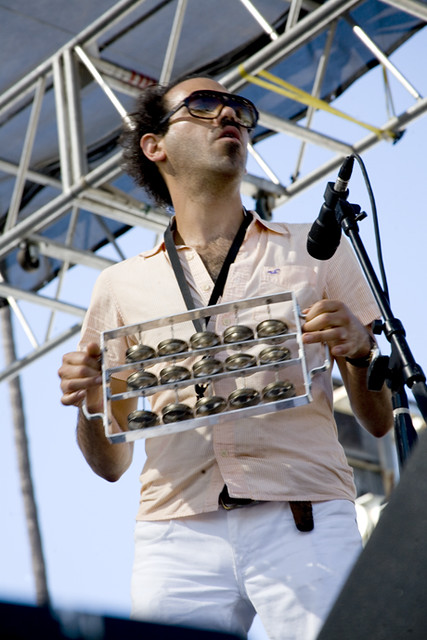In a vibrant daytime photograph, a man, possibly of Filipino descent, stands front and center on a large open-air stage. The setting is bright with clear blue skies visible around the steel girders and scaffolding that form the stage's roof. He appears to be in a concert setting, captured from the perspective of the audience.

The man is dressed in a peach short-sleeved shirt, white pants, and a black belt. His appearance is notable with dark curly hair that is thinning at the top, large dark sunglasses, a small moustache, and designer stubble. He has a slightly open mouth and pink lips. His chest appears hairy in the open-neck shirt.

He holds a unique rectangular musical instrument in front of him featuring three rows of five small symbols, each no more than two inches in diameter. The instrument has handles on either side, suggesting it might be shaken to create sound. A microphone stand is positioned towards the instrument, indicating he is performing rather than singing. The image is sharply focused, capturing the dynamic energy and detail of the live performance scene.